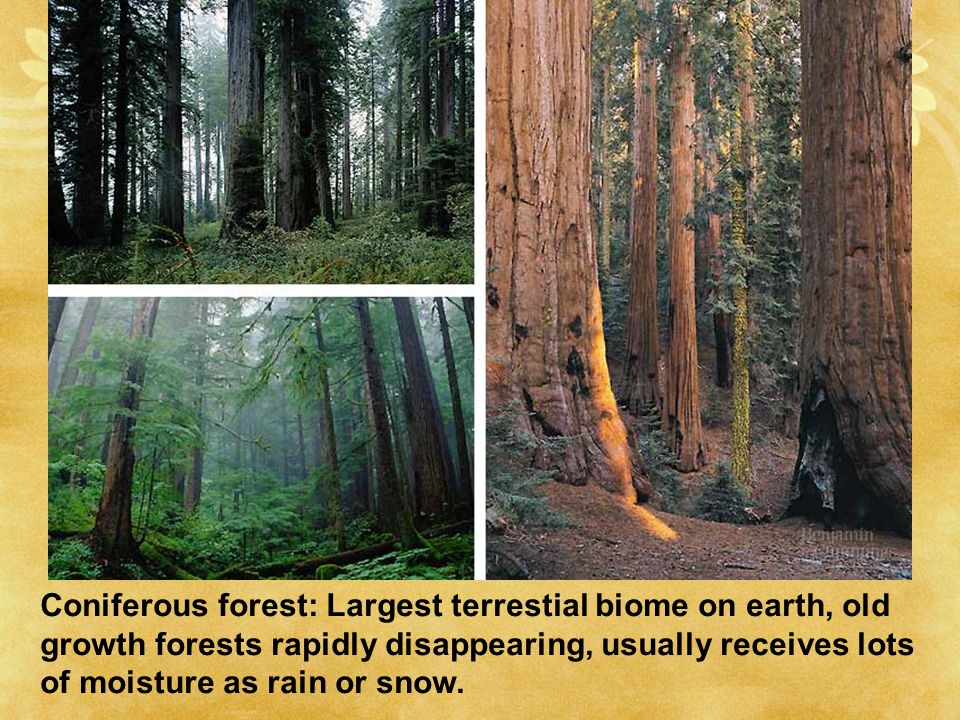The image comprises a composite of three separate pictures of forests, arranged on a yellow background possibly adorned with flower petals. The photograph on the right dominates with its depiction of what appear to be towering redwoods, characterized by their large trunks and clear, sunny weather. On the left, the top picture shows a darker forest scene with some greenery at the bottom, while the lower left image is lighter with denser vegetation and a misty atmosphere. These left-side images also feature large trees and a noticeable presence of green foliage. Below the collage, in black text, the caption reads: "Coniferous forest, largest terrestrial biome on Earth, old growth forest rapidly disappearing, usually receives lots of moisture as rain or snow." This suggests the images are part of an educational display highlighting the attributes and environmental concerns of coniferous forests.